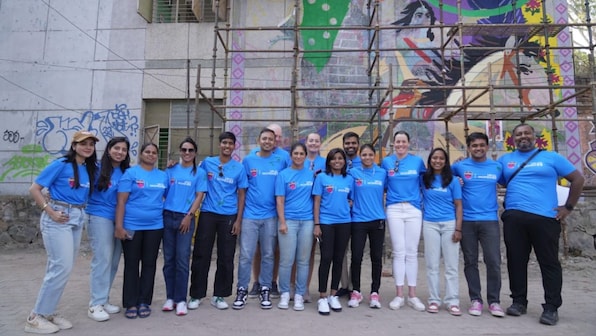This photograph captures a lively group of approximately 15 young adults standing outside a graffiti-covered urban building in India, possibly during a company retreat. They are all wearing matching bright blue t-shirts adorned with some unreadable white text and a shield-like logo on the breast area. The group is arranged in a line on a gray, possibly tiled surface, with a few people positioned slightly behind the main row. Most of them are dressed casually, pairing their t-shirts with various pants and sneakers, and they are all smiling. The building behind them features a mix of scaffolding, artwork, and graffiti, adding an interesting contrast to the cheerful atmosphere of the group.